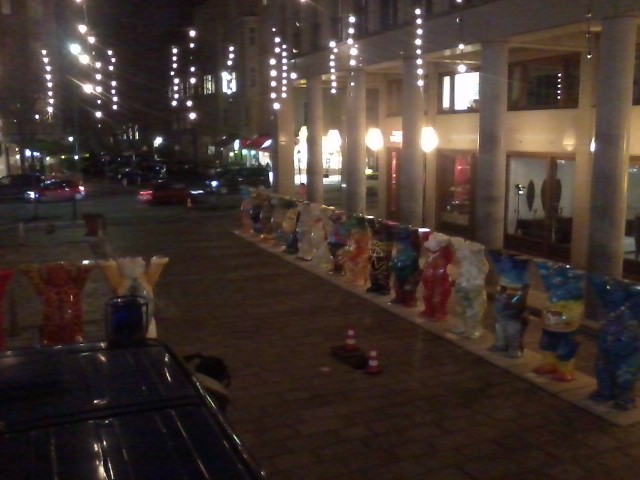The image captures a dimly lit city street at night, featuring a row of statues or figurines aligned along a sidewalk. The statues depict bear-like figures, each adorned with various colors including blue, yellow, red, white, and black, though the exact patterns are indistinct. They appear to represent different cities or countries, facing different directions towards the street and storefronts. The street itself shows multiple cars with illuminated lights, although their colors are difficult to discern due to the blurriness. Some of the cars seem to be in motion. In the scene closer to the viewer, there are illuminated columns of a nearby building, and several windows casting a soft glow. A black car with possibly a blue light on top is partially visible to the left, and in the middle of the street, there's a hole or manhole marked by two industrial cones. The overall composition of the image suggests a lively but obscured urban setting with multiple light sources and indistinct figures creating a mysterious night-time cityscape.